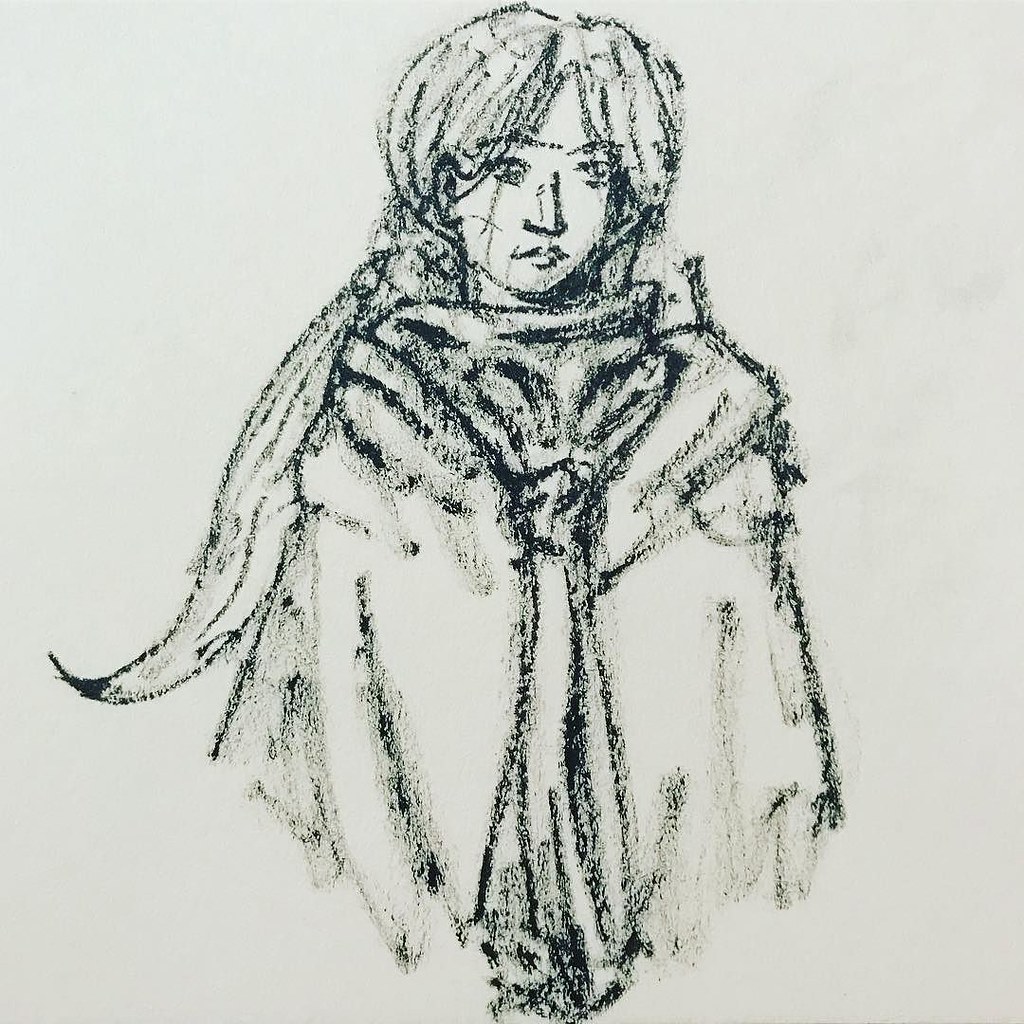The image depicts a detailed pencil or charcoal sketch on an off-white, slightly grayish sheet of paper. The sketch features a young woman with long hair styled in a braid that extends past her torso, with bangs framing her face and revealing a bit of her forehead. She is dressed in a billowy, non-form-fitting cloak or robe, which wraps around her entire upper body, obscuring her arms and hands. In addition, a scarf is draped down the center of her chest. The artwork is rendered entirely in shades of black, white, and gray, capturing the figure from the waist up, facing towards the viewer.